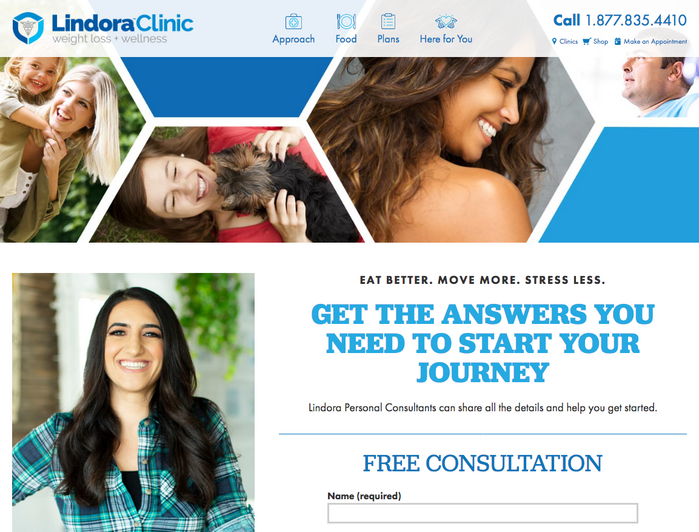The image is a screenshot of an advertisement for the Lindora Clinic, a weight loss and wellness center, prominently positioned in the upper left-hand corner within a white banner. The clinic's logo, featuring a shield icon in three shades of blue, is accompanied by the text "Lindora Clinic" in navy blue and sky blue, followed by "Weight Loss + Wellness" in gray font.

To the right, bold blue text reads, "Approach Food Plans" with a call to action: "Here for you. Call 1-877-835-4410." Additional service options, "Clinics," "Shop," and "Make an Appointment," are listed below this.

The advertisement features images of several individuals:
- A young mother with blonde hair playfully carrying a young girl on her back.
- A young woman with brown hair relaxing with a dog that has dark brown and black fur.
- Another woman with brown, wavy hair standing alongside a man with short brown hair.
- Below these, a smiling woman with long brown hair in a green flannel shirt is highlighted.

Next to the smiling woman, motivational text encourages viewers to "Eat Better, Move More, Stress Less." It invites potential clients to "Get the answers you need to start your journey," with a promotional message promoting free consultations with Lindora professional consultants. The phrase "Name Required" is noted, possibly indicating a sign-up requirement for the free consultation offer.